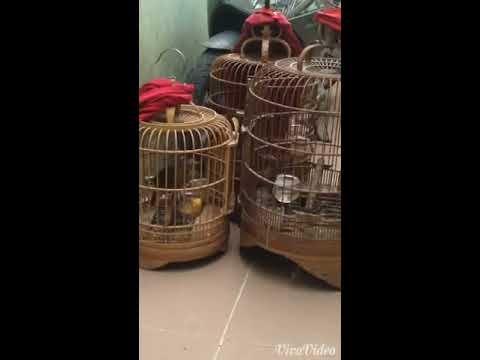This photograph features three antique-style bird cages, arranged on what appears to be a beige or sand-colored tiled floor. The image is framed by two narrow, vertical black panels on the left and right sides. The central panel, which is wider, showcases all three bird cages that vary in size; a smaller cage on the left, a medium-sized one partially visible at the back, and a taller cage on the right.

Each bird cage is round with curved tops and has a red cloth or rag wrapped around the hook area for hanging. The cages, likely made of brass or painted golden, evoke a style that might date back to the 1940s due to their simplicity and non-mass-produced appearance. Within the smallest cage on the left, a yellow bird can be observed, though its details are indistinct. The right cage also appears to have a bird and includes a crystal bowl at the bottom, possibly for water. The background consists of a pale teal blue wall accented with black, contributing to the overall vintage aesthetic of the scene.